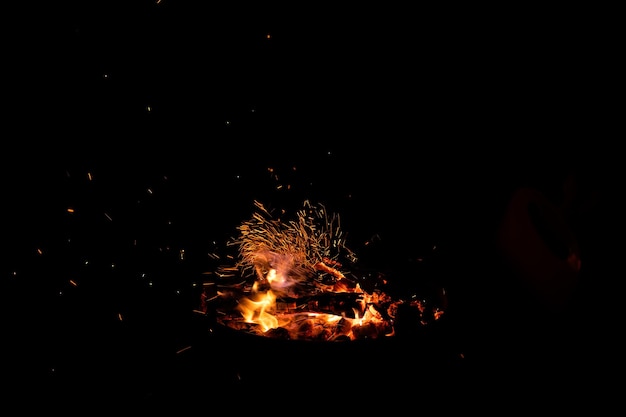The landscape-oriented color photograph captures a dramatic night scene dominated by darkness, with the only source of light being a fiery spectacle in the center near the bottom. The fire takes on a molten appearance, resembling a large fire without the typical blazing flames. Instead, fiery sparks shoot outwards, bending to the left as if blown by the wind. A prominent black piece of wood or indiscernible object is pressed against the molten core, from which these sparks seem to originate. Surrounding this central fire are shapes that could be people or simply rocks and wood arranged in a way that mimics human outlines, shrouded in the darkness. The sparks create a spattering of light near the top left of the image, adding to the dynamic, fiery effect. The photograph is a representation of realism, capturing the raw and mesmerizing beauty of a fire against a backdrop of deep night.